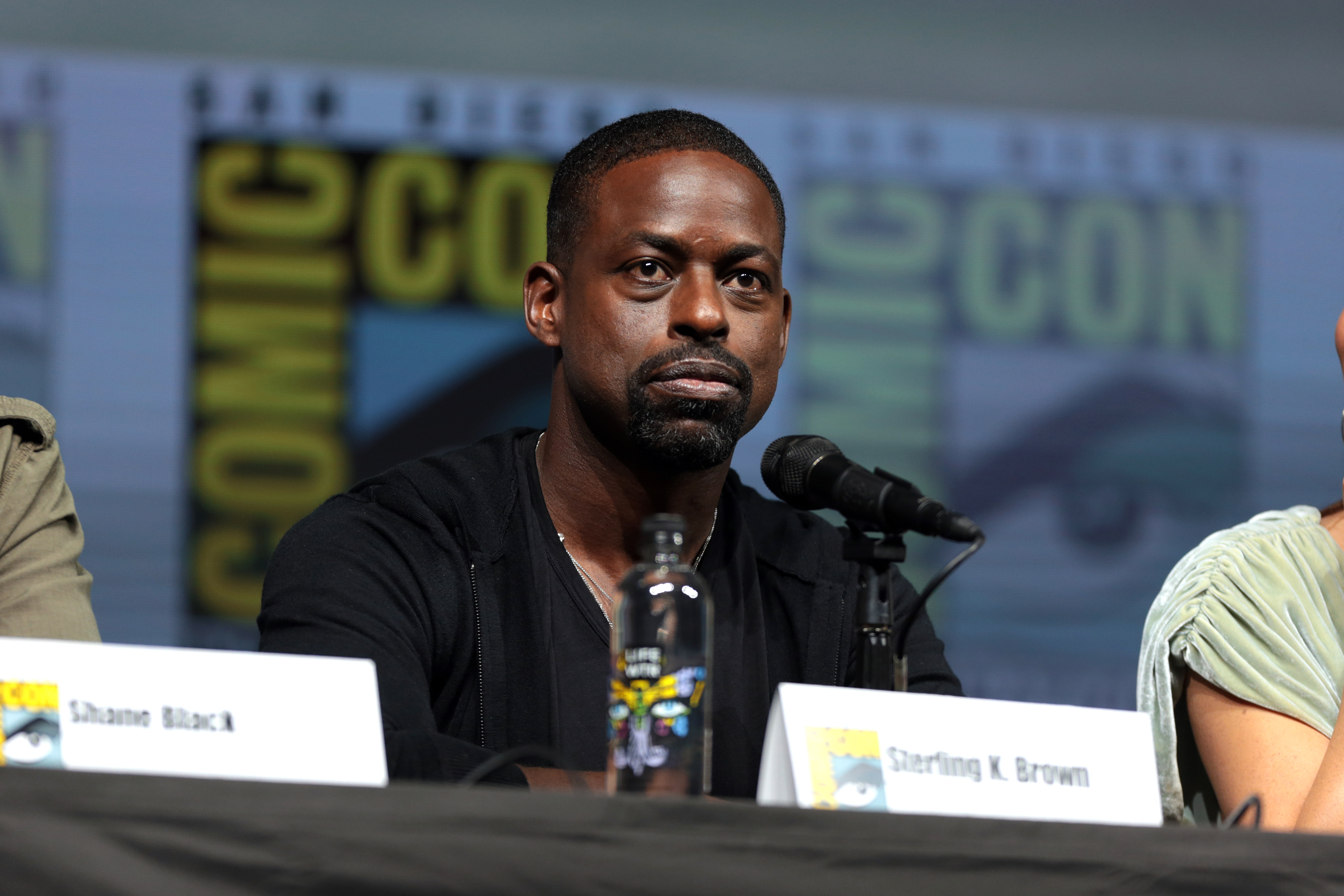In the image, Sterling K. Brown is the central figure, a black man with short black hair, a mustache, and a closely shaven goatee. He wears a dark-colored jacket over a black shirt, enhanced by a visible chain around his neck. Seated at a table, he is intently focused on something out of the frame, with a neutral expression. He is positioned behind a microphone, with a water bottle and a name placard in front of him, confirming his identity as Sterling K. Brown. Flanking him are two indistinct individuals; on his right, an arm is visible, clad in a short-sleeved greenish-silver shirt, belonging to a white person, and on his left, another partial arm covered in a gray shirt. Behind them, the backdrop features multiple Comic Con signs with a distinctive eye design, set against a greenish background, adding context to the scene. At the very bottom of the image, the table appears to be covered by a gray cloth.